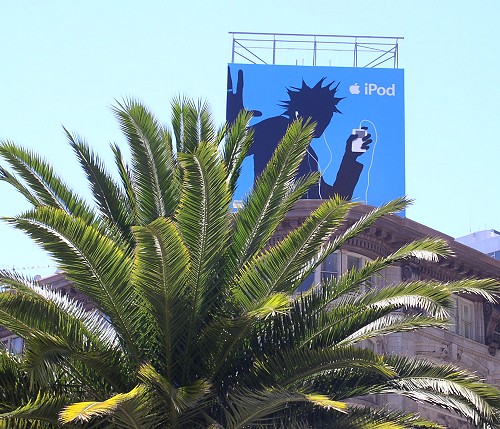A striking photograph captures the architectural grandeur of an arena from the ground up, emphasizing its intricate details. Dominating the foreground is a lush palm tree, its abundant green fronds juxtaposed against the sleek, gray building behind it. The building features a protruding overhang adorned with a classic Greek key design just beneath its eave. Further enhancing the structure's elegance are the neatly paned windows encapsulated by the ornate overhang. Atop the building, a silver scaffolding supports a vibrant banner. The banner, set against a blue background, showcases the silhouette of a person with spiked hair energetically dancing, holding a white iPod in their left hand. The device's cord winds up to white earphones in the dancer's ears. The top right corner of the banner prominently displays Apple's iconic logo alongside the word 'iPod.' This entire scene unfolds against the backdrop of a serene, light blue sky.